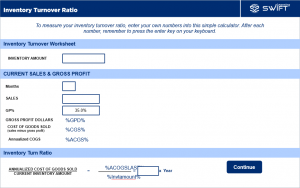In this image, at first glance, details are challenging to discern due to its small size. Starting at the very top, there is a narrow dark blue rectangle. In the top-left corner of this rectangle, three words, "Inventory Turnover Ratio," are clearly written in white text. On the top-right corner, the word "SWIFT" is visibly displayed, accompanied by what seems to be their company logo to the left, both also in white text.

Below this top section, against a white background, there appear to be additional words which look slightly blurred and are rendered in light blue text. Spanning horizontally across the middle of the image is a large sky-blue rectangle. Positioned within this rectangle is the phrase "Inventory Turnover Worksheet" written in dark blue text.

Continuing downward, we encounter another white background area populated with dark black text. Further below, another section marked by a sky-blue rectangle emerges, this one bearing the inscription "Current Sales and Gross Profits" in dark blue text. Finally, at the bottom-right corner, a dark blue rectangle with the white text "Coronavirus" is present, while at the bottom-left, some black text is visible. Additionally, the phrase "Inventory Turn Ratio" in dark blue writing is positioned above this text.